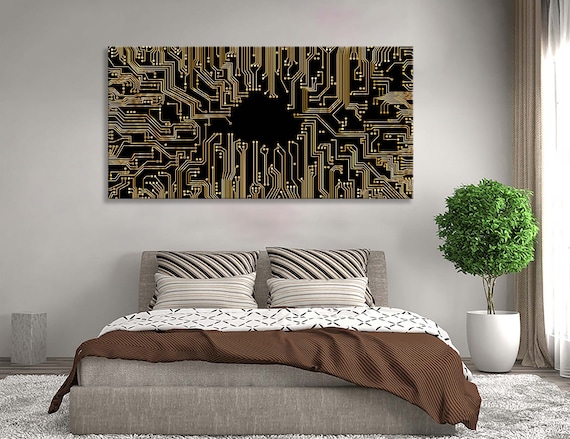This photograph captures a well-coordinated bedroom with a modern touch. Dominating the floor is a large, white fuzzy rug upon which a gray linen platform bed is carefully positioned. The bed features a neatly folded dark brown coverlet, with a contrasting patterned cover peeking out by the pillows. The pillows themselves showcase a harmonious blend of horizontal stripes in shades of brown, tan, and gray. Behind these striped pillows are larger dark brown and gray throw pillows, adding an extra layer of texture and comfort.

Adjacent to the bed on the right side stands a potted plant, characterized by its thin brown stems and round, bushy green leaves, all housed in a sleek white ceramic pot. The gray walls provide a neutral backdrop for this verdant touch.

Above the bed, a large, rectangular piece of artwork commands attention. This striking poster features intricate designs reminiscent of a circuit board, with a black background and an array of gold and white lines radiating from a central point. This captivating piece not only enhances the modern aesthetic of the space but also adds an intriguing focal point.

To the right of the scene, a window framed by lightly illuminated curtains hints at a sunny day outside, casting soft light that further accentuates the room's sophisticated blend of brown tones and contemporary details.